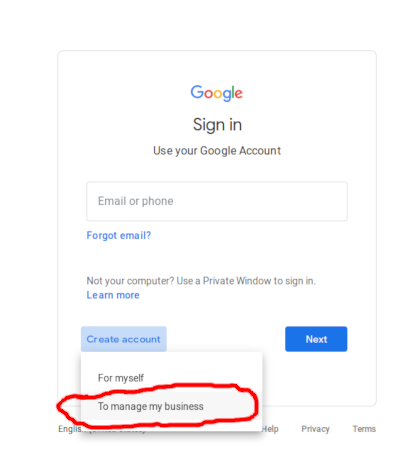This is a detailed screenshot of a pop-up on a website with a white background. The main portion of the pop-up features a thin light gray outline with rounded corners, giving it a sleek and modern look. At the top center of the pop-up is the recognizable multicolored Google logo.

Directly below the logo, large black centered text reads "Sign in," followed by smaller black centered text that says "Use your Google Account." Further down, after a line break, there is a text entry box with a thin light gray outline and slightly rounded corners, containing placeholder light gray text that reads "Email or phone."

Under the text entry box, on the left side, blue text reads "Forgot email?" Two line breaks below this, small light gray text says, "Not your computer? Use a private window to sign in." Below this on the left side, blue text reads "Learn more."

Towards the bottom of the pop-up, there is a light blue button with dark blue text that reads "Create account." To the right of this button is a dark medium blue button with white text in the middle that reads "Next."

Attached to the "Create account" button is a descending white pop-up window, perfectly aligned on the left side with the button. This secondary pop-up casts a light gray shadow behind it, adding depth. It contains two lines of medium gray text: "For myself" and "To manage a business," with the second option highlighted within a light gray rectangle and circled by an irregular red outline.

Beneath this drop-down menu, partially obscured by the secondary pop-up, there are additional lines of medium gray text, providing further information.